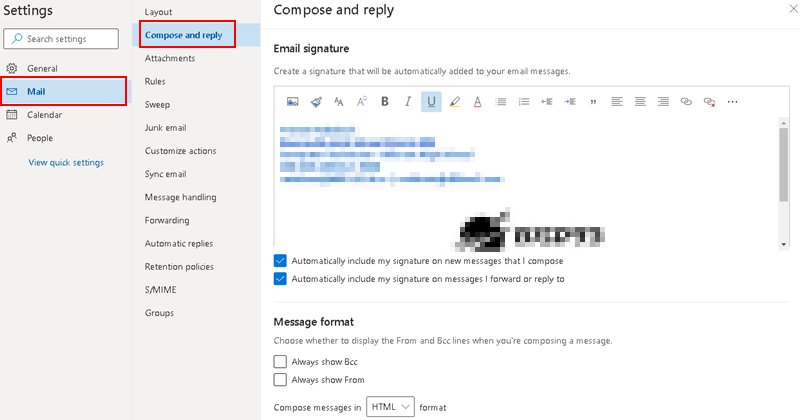The image depicts an educational interface likely designed for learning purposes. The background is composed of a gray hue, setting a neutral tone. On the left side, there are various settings options. The first row under the settings title features a search bar labeled "Search settings." Below the search bar, a menu lists several categories: General, Mail, Calendar, People, and View quick settings.

The "Mail" category is highlighted in blue text, standing out against the otherwise gray background. A red triangle is drawn around the highlighted Mail category, suggesting emphasis.

To the right, another column presents further options, arranged vertically: Layout, Compose and reply, Attachments, Rules, Sweep, Junk email, Customize actions, Sync email, Message handling, Forwarding, Automatic replies, Retention policies, eSports, MIME and groups. The "Compose and reply" option is also in blue, with a red triangle framing it, similar to the Mail category.

The selected "Compose and reply" section details instructions for creating an email signature. It states, "Create a signature that will be automatically added to your email message." The text area intended for the email signature includes blurred lines of blue text and a partially visible blue logo, indicting sensitive information. The word processing toolbar appears at the top of this section.

At the bottom of the text area, two options are ticked: "Automatically include my signature on new messages that I compose" and "Automatically include my signature on messages I forward or reply to." Below these options, the interface offers additional formatting choices, indicated by the partially visible word "create."